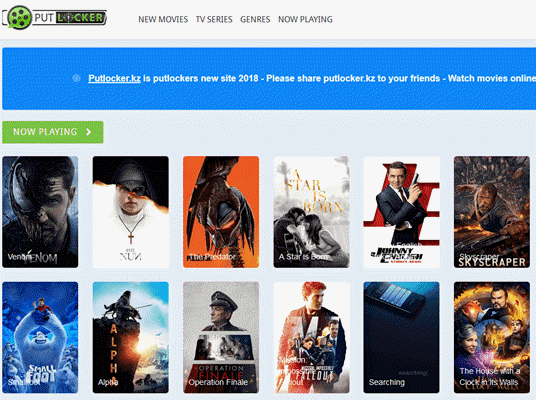The image depicts a movie website named "PuttBlocker." The website’s name is displayed prominently at the top left, accompanied by a logo featuring a green circular background with five smaller circles. To the right of the logo, four categories are listed: "New Movies," "TV Series," "Genres," and "Now Playing."

Below the navigation bar, a blue rectangular banner announces, "PuttBlocker is New site 2018," urging users to share the website (puttblocker.kz) with their friends and to "Watch movies online."

The section beneath this banner showcases several movie covers under a "Now Playing" label highlighted in a green rectangle. The top row features six movies from left to right: "Venom," "The Nun," "Predator," "A Star is Born," "Johnny English," and "Skyscraper." The second row begins with a movie related to snow, followed by "Alpha," "Operation Finale," "Mission Impossible," "Searching," and "The House with a Clock."